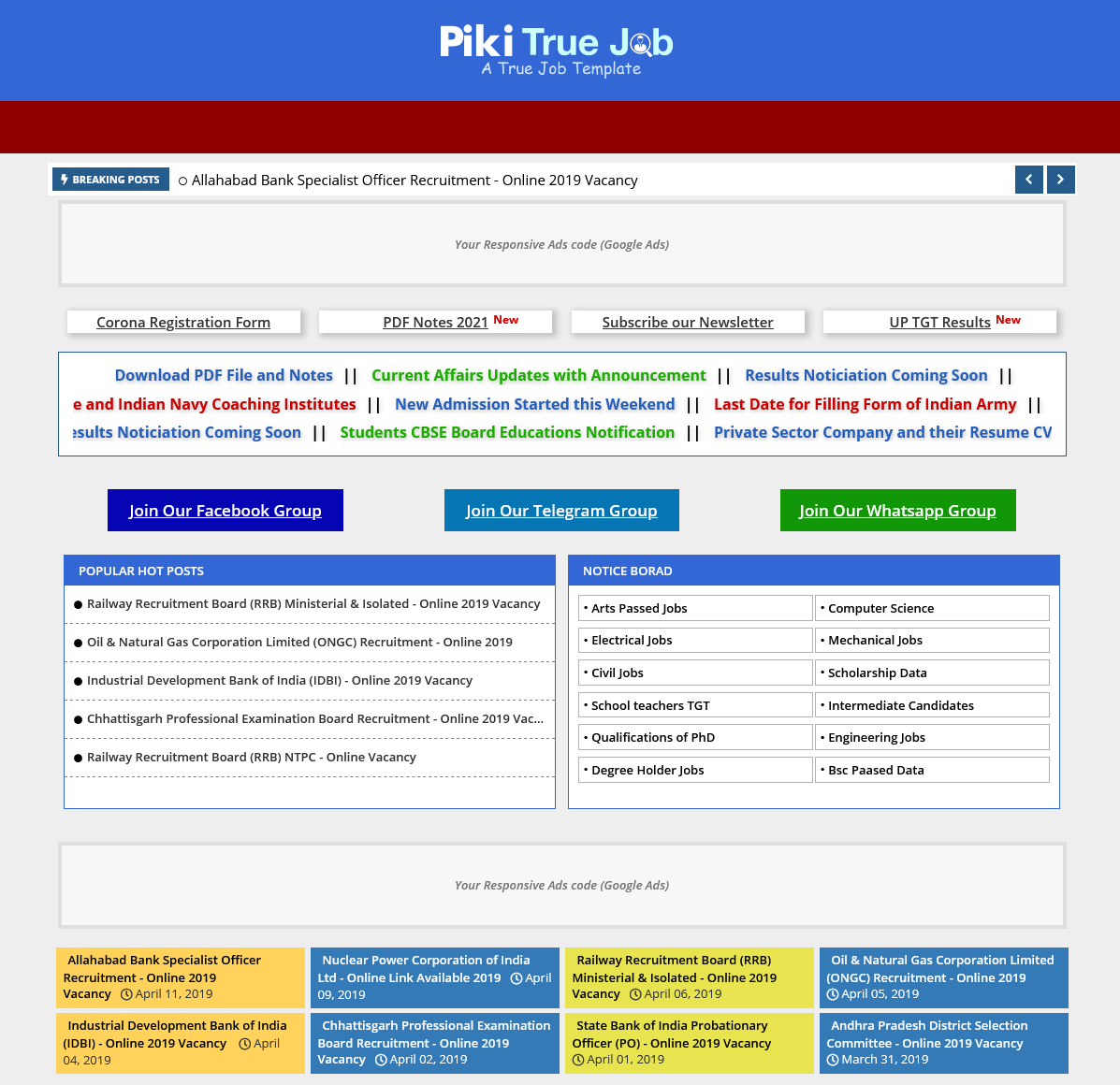At the top of the image, there is a long blue rectangle featuring text in white and blue. The text begins with the word "PIKI" in white, followed by the word "true" in blue, and the word "job" in white, with the 'O' replaced by a large white circle. Beneath this, the phrase "True Job Template" is displayed prominently. Below the header, various options are presented:

1. A green option to download a PDF file and notes titled "Current Affairs with Announcement."
2. A blue option stating "Results Notification Coming Soon."
3. A red option for the "Indian Navy Coaching Institution."
4. A blue notice indicating "New Admission Started This Weekend."
5. An option for "Private Sector Company and Their Resume/CV."

Further down, there are three horizontally aligned rectangles:
1. A dark blue rectangle with the text "Join the Facebook Group."
2. A blue rectangle encouraging users to "Join Our Telegram Group."
3. A green rectangle prompting users to "Join Our WhatsApp Group."

Near the bottom, a series of differently colored squares are visible. From left to right, they include a dark yellow square, a blue square, a lighter yellow square, and another blue square. Above these squares, there is a "Notice Board" and a "Popular Hot Posts" board.